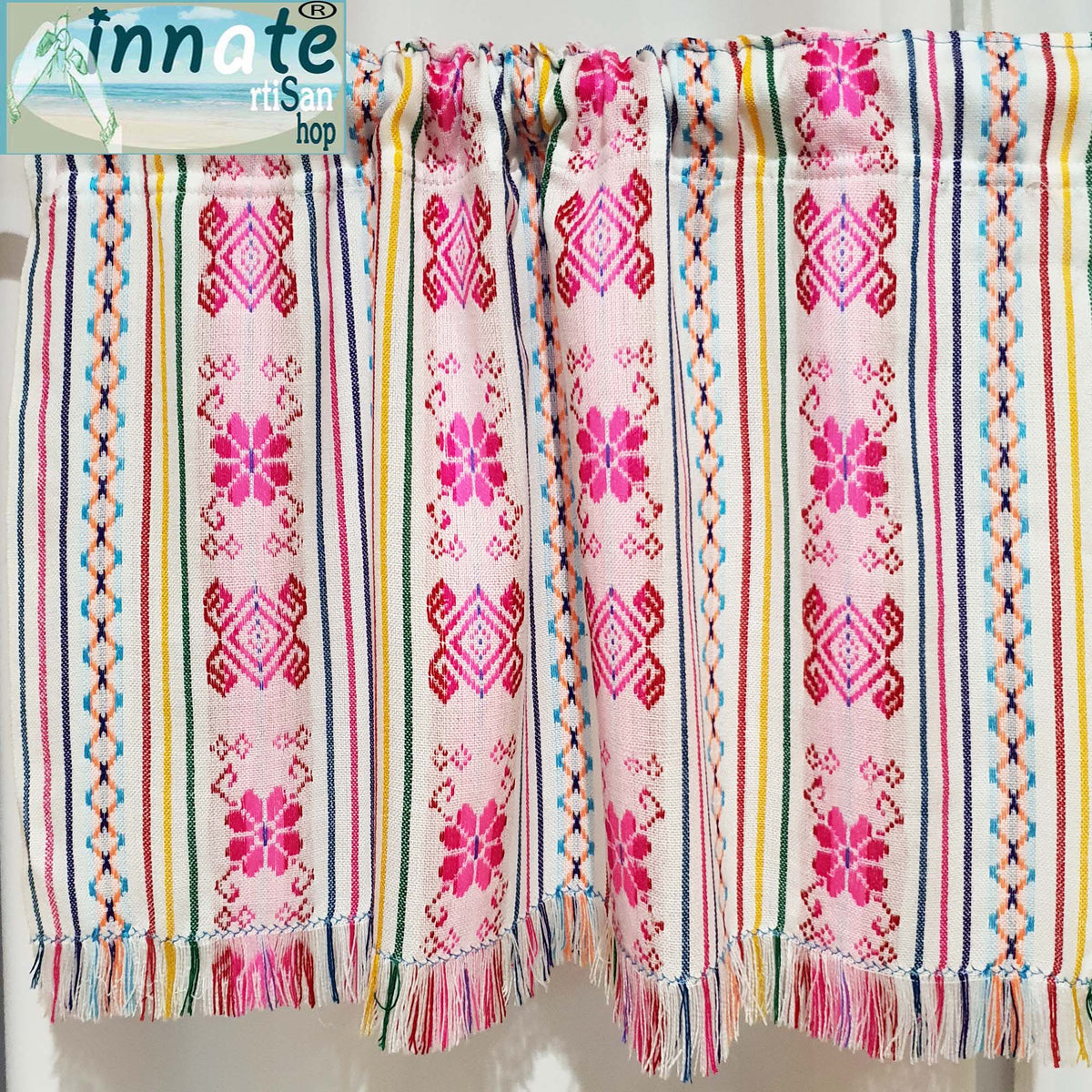This photograph features a window curtain that dominates the frame, likely designed for a shorter window. The curtain is composed of two sections of thick fabric with a vertical pattern featuring alternating designs. Specifically, the fabric showcases white diamond shapes interspersed with pink flowers and intricate designs, separated by vertical lines in shades of gray and reddish hues. The bottom of the curtain has a loose-thread border, adding a casual, decorative touch. At the top of the image, the company's logo "Innate RTI Sand Shop" is visible, featuring a beach scene with an ocean backdrop and a pair of hands crafting an item, possibly green leaves, against the background. The logo text uses a mix of black and white fonts.